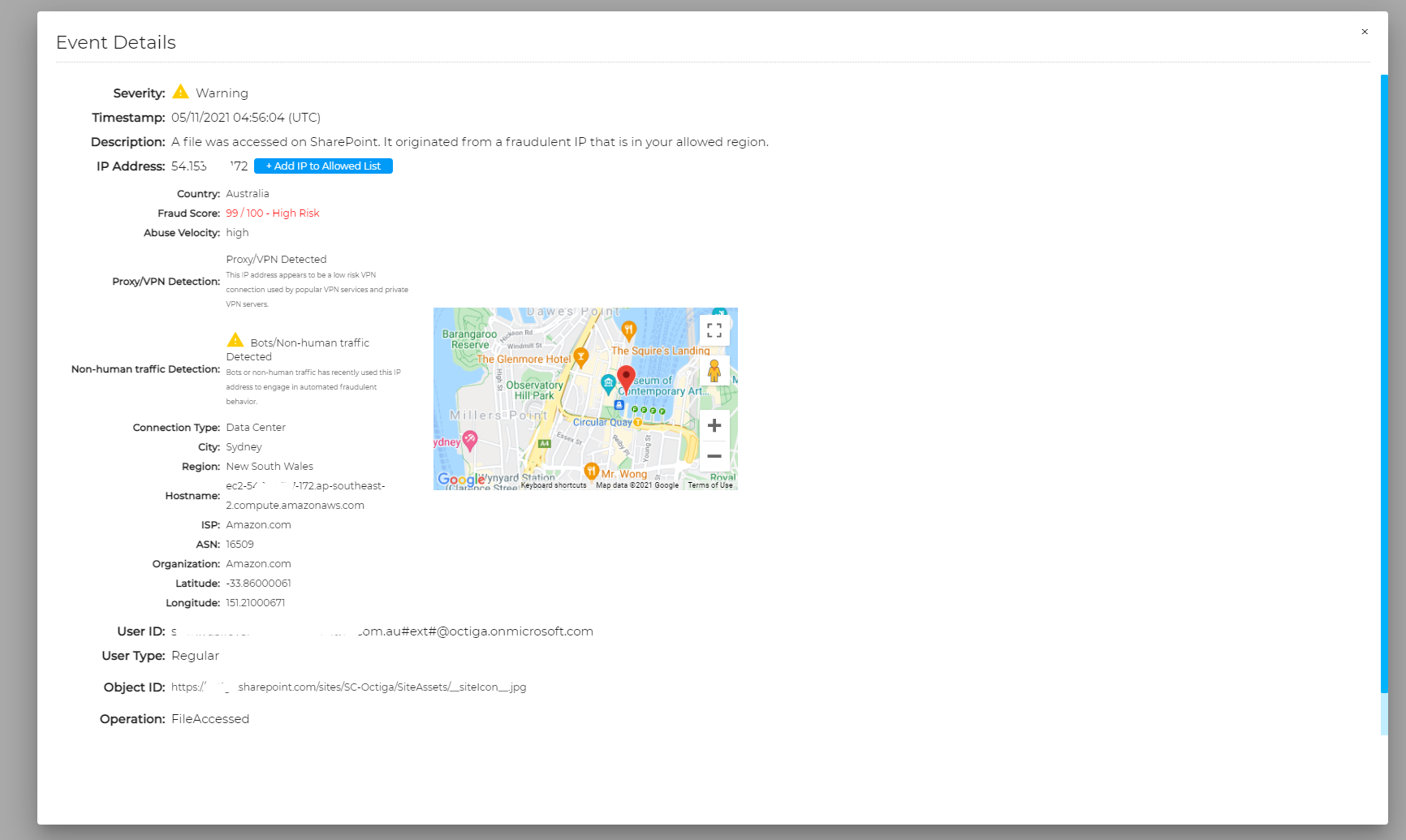The image is a rectangular screenshot meticulously detailing an event's information. Positioned on the left side of the image, in dark gray text, is a header labeled "Event Details." Directly below this header, there are various warnings and pieces of information, including numerous timestamps documenting the progression of the event.

Dominating the center of the image is a map, identified as an excerpt from Google Maps, with the recognizable Google logo in the bottom left corner. The logo itself is displayed in vibrant shades of blue, red, yellow, green, and another red. The map highlights a city area surrounded by blue, which likely represents water. Various icons populate the map, including symbols for a hotel and several restaurants.

On the left side of the image, accompanying the event details, is a comprehensive list of event occurrences. This list includes severity levels, timestamps, descriptions, IP addresses, non-human traffic detections, connection types, cities, regions, hostnames, ISPs, user IDs, user types, object IDs, and operations.

The image features a white background bordered by a medium gray margin, framing the detailed information concisely and neatly.